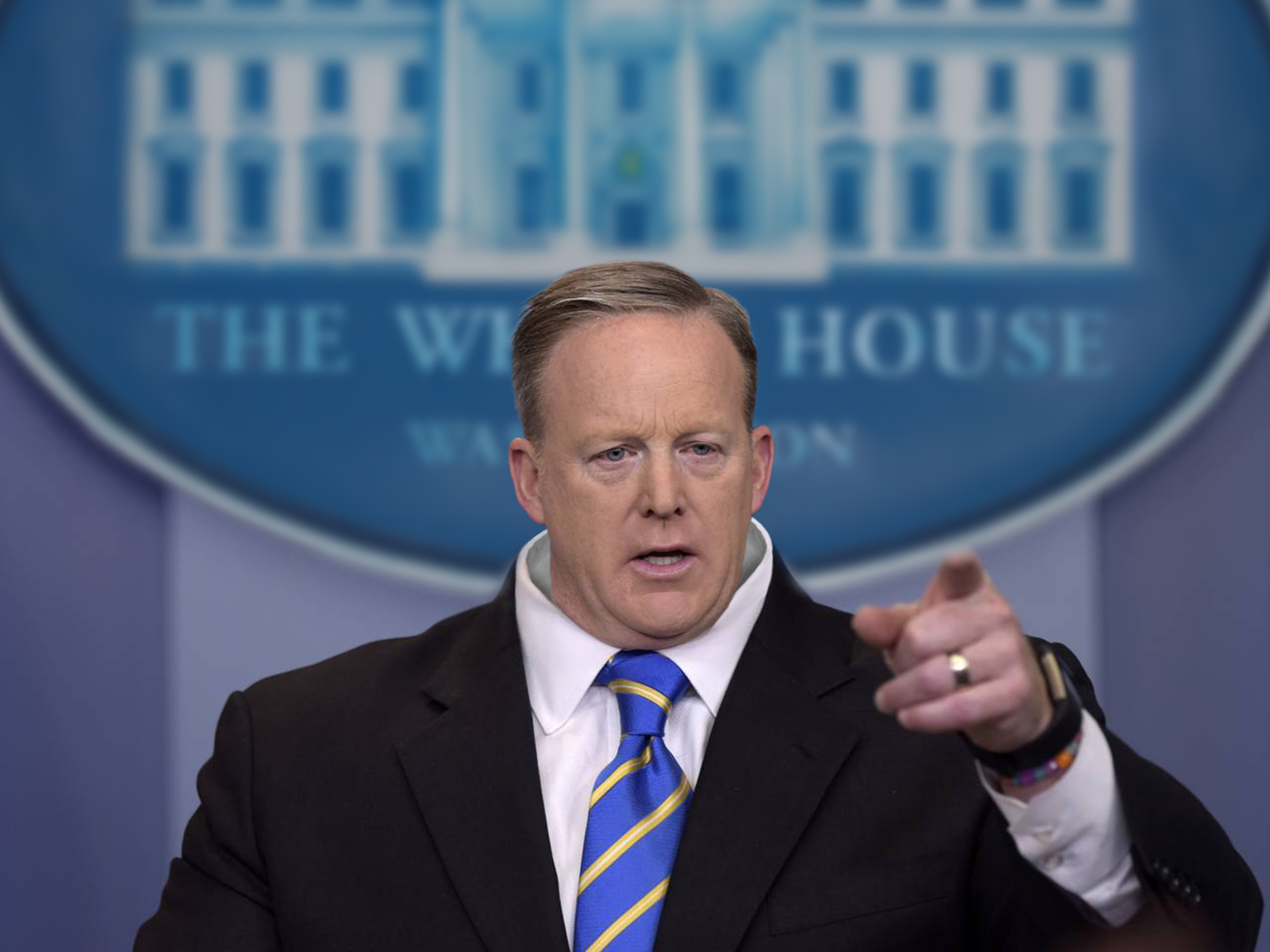The image depicts a Caucasian man, one of the former Speakers of the House during Donald Trump's presidency, standing and speaking at what appears to be the White House. He has short gray hair, blue eyes, and is wearing a black suit, a blue tie with yellow diagonal gold lines, and a white dress shirt. His left hand, which bears a wedding band, is extended and pointing out towards the audience. Additionally, he is wearing a smartwatch and a beaded bracelet, possibly made by a child. Behind him, there's a backdrop with an oval-shaped logo featuring an illustration of the White House, partially obscured by his head, contributing to an overall comical effect, as his head appears disproportionally small for the suit. This gives the impression that the image may be photoshopped. The setting seems to be an indoor conference or seminar, though it's unclear whether it's daytime or nighttime.